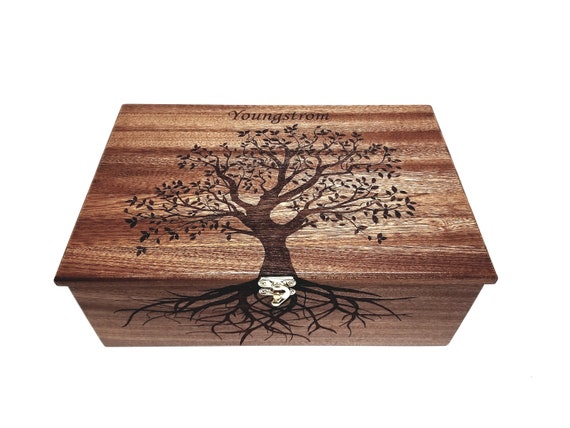This photograph features an ornately crafted wooden box, predominantly showcasing its top and front sides. Engraved on the lid is the name "Jungstrom," meticulously spelled Y-O-U-N-G-S-T-R-O-M. Dominating the lid is a striking design of a tree, which appears to be either carved or burnt into the wood. The tree's trunk extends upward into a network of branches and leaves, forming a half-spherical, tree-of-life pattern. The wood itself is laminated, with the tree design rendered in a darker tone to stand out against the lighter stained and finely finished grain of the box. At the base of the tree, where the lid meets the front of the box, there is a silver lock mechanism. Below this latch, extending onto the front of the box, the tree's roots are painted in black, fanning out in a circular fashion to symbolize the depth and strength of its roots. The box is rectangular in shape, combining intricate artistic details with a simple, elegant form.